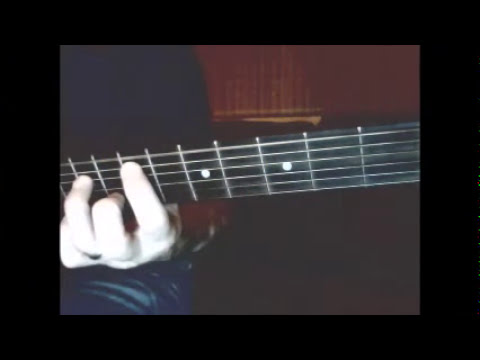In this close-up image, a person is captured playing a guitar in a dimly lit indoor setting. Positioned on the left side, only parts of the individual are visible: the left torso and upper chest, left leg clad in blue jeans, and the left arm and hand actively playing the guitar. Their shirt appears to be dark blue with a dark red sleeve. The left hand of the person, whose complexion suggests they are Caucasian, is prominently featured, with the first and third fingers curled in a chord position while the middle and ring fingers extend along the guitar strings. The visible part of the guitar includes the fretboard and the black neck extended horizontally across the image with a slight incline to the right. The background is a rich wooden hue, resembling redwood, and the image is framed by a black border. The overall tone of the photo has a sepia-like warmth, and there is no text present anywhere within the image.